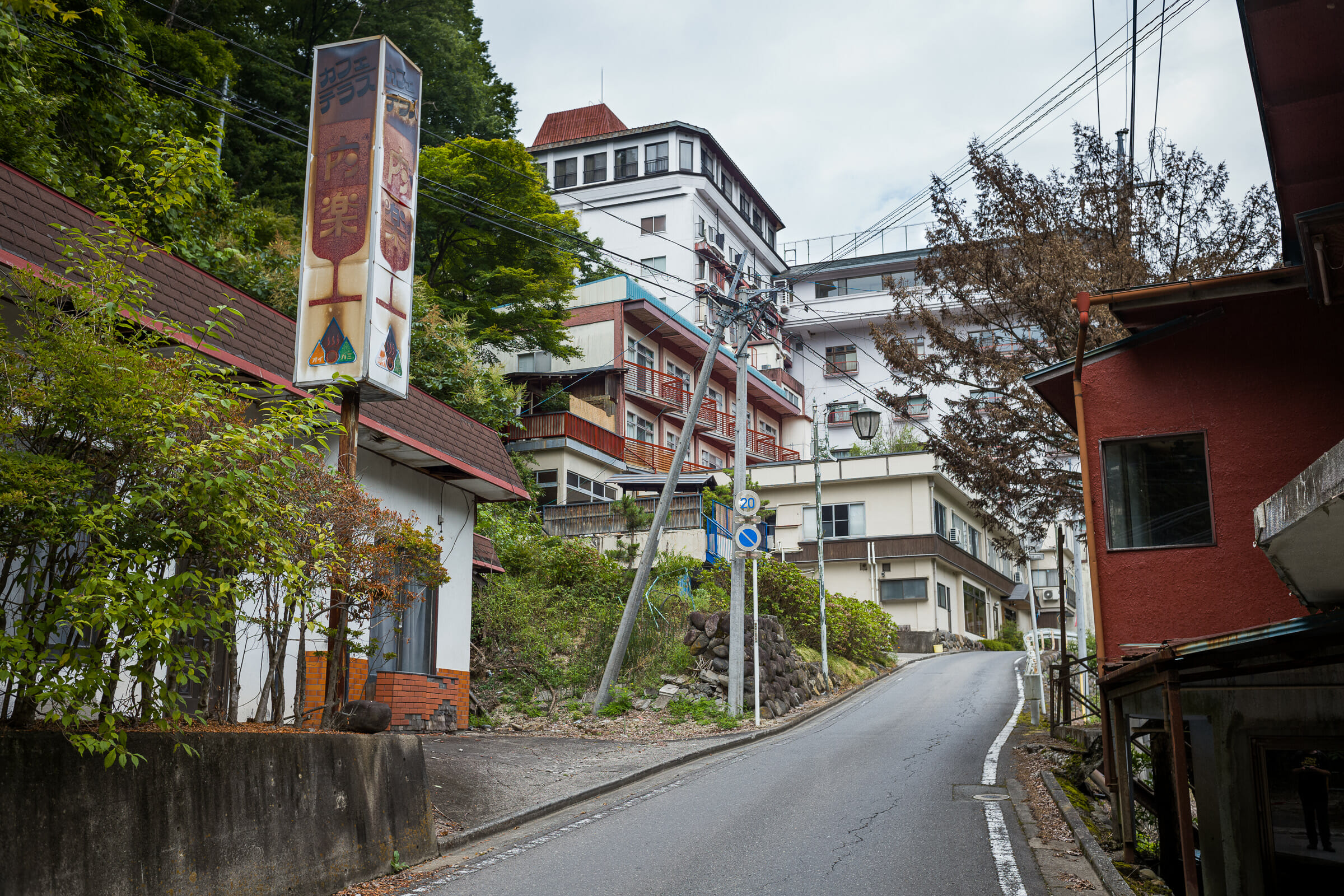The image depicts a slightly gloomy day in a small city or town with a narrow, one-way street bordered by white striped lines. The street ascends a hill and is flanked by various buildings on either side. On the left side, there's what seems to be a business establishment, accompanied by a wooden fence and an area with trees. The building appears to have multiple stories, possibly with separate patios, and extends up to eight stories. In the foreground, on the right, is a distinct red building with a brown base, alongside more trees and utility poles with low-hanging wires. Various street signs are present, including a blue circular sign with a line through it and a blue sign indicating a 20-speed limit. The skyline in the background features larger white buildings with red roofs. Overall, the sky appears grayish-blue with numerous clouds, adding to the slightly overcast ambiance of the scene. Notably, the text on the signage is not in English, suggesting an international location. The street scene is devoid of vehicles and people, contributing to its tranquil, somewhat somber mood.